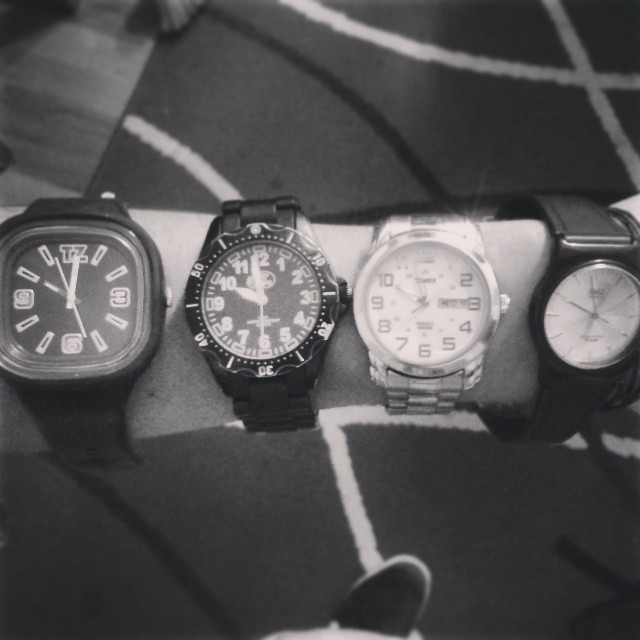This black and white close-up image showcases a person's thin arm adorned with four distinct analog wristwatches. The arm is prominently hair-free, with either a slight shine or faint hair visible on the upper right part. The orientation of the arm is unclear due to the close-up nature of the photo, which focuses on the watches. Below the arm, a black shoe with a white trim slightly points towards the right, resting on a multicolored carpet that appears primarily gray with white and black arcing lines in the grayscale image. An area that might be a wooden floor is faintly visible in the upper left of the frame.

Starting from the left, the first watch features a dark band and a rounded square face. Instead of a '12', it reads 'TZ', with only the numbers 3, 6, and 9 visible amidst a deeper bezel. Next is a sportier watch with a standard analog face and rotating outer dial, showing numbers 10, 20, 30, 40, and 50 on the scale. The third watch in line has a stainless steel band; it displays all the numbers, though 1, 11, and 12 are partially obscured by lighting. The final watch on the right, with a solid black plastic band, showcases a minimalist design with mark indicators instead of numbers.